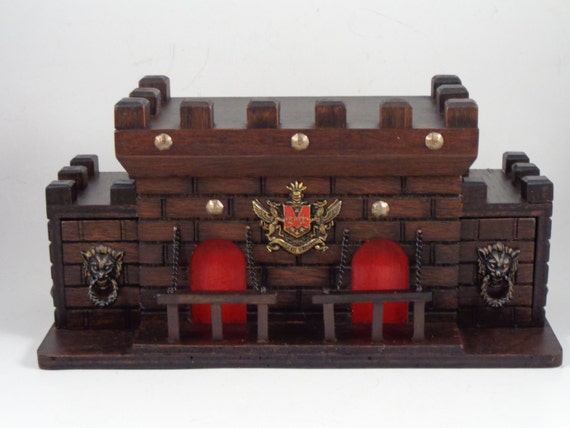The image showcases an intricately crafted wooden figurine set on a thin, dark wooden base. The base is comprised of a thinner layer at the bottom. Rising from this foundation is a central, elevated wooden panel, mirroring the structure below. The composition features two small, chamber-like sections adorned with a horizontal wooden beam intersected by three vertical beams—one each at the ends and one in the center. Behind these beams, a vivid red flame appears, emanating from the central space.

Between the two archways with the flames, a coat of arms is prominently displayed, guarded by two metallic, animal-like creatures that resemble angelic figures. In the heart of the coat of arms, an ornate letter 'M' is carved. Above this, another wooden panel supports a central creature figurine, set against a wooden backdrop.

On each side of the central panel, lower protrusions are adorned with lion heads, each featuring a knocker, akin to traditional door knockers. The upper portion of the figurine flattens at the center but is flanked by thicker, square components—three on the back panel, three on each side, and four prominently positioned in the center. The entire piece radiates a sense of gothic elegance and meticulous craftsmanship.